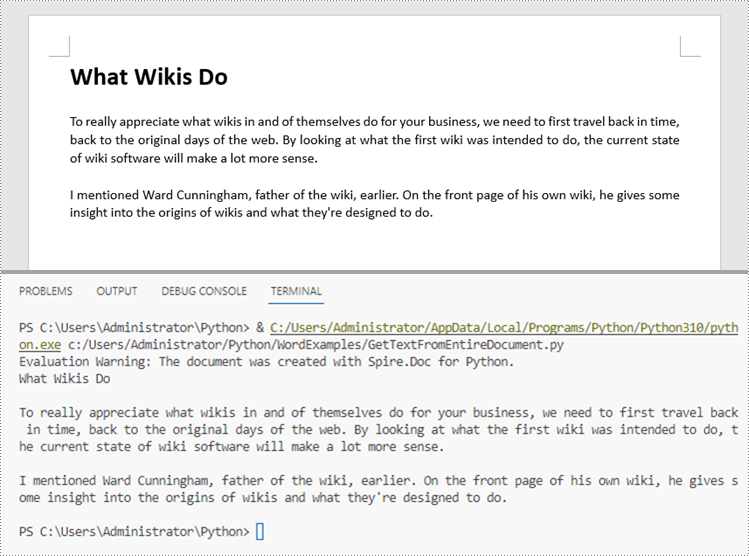Screenshot of a Wiki Page with Code Implementation

In this screenshot, we see an informative page discussing the functionality and historical background of wikis. The text explains the significance of wikis for businesses by taking a trip down memory lane, highlighting the original intent behind their development. It references Ward Cunningham, known as the father of the wiki, and sheds light on his insights about the origins and purpose of wikis as outlined on his own wiki's front page.

Beneath this explanatory text, four different tabs are visible: Problems, Output, Debug Console, and Terminal, with the Terminal tab underlined, indicating it’s currently selected. The terminal displays a segment of Python code, which essentially translates the descriptive content about wikis into a coded format. 

At the bottom of the terminal, there is a command-line input showing the path “PS C:\Users\administrator\Python>,” implying that an administrator is executing or editing the code.

This setup illustrates not only the theoretical explanations of wikis but also provides a practical example of what wikis do, by converting the descriptive text into a Python script, offering a comprehensive understanding from both a user and an administrator's perspective.